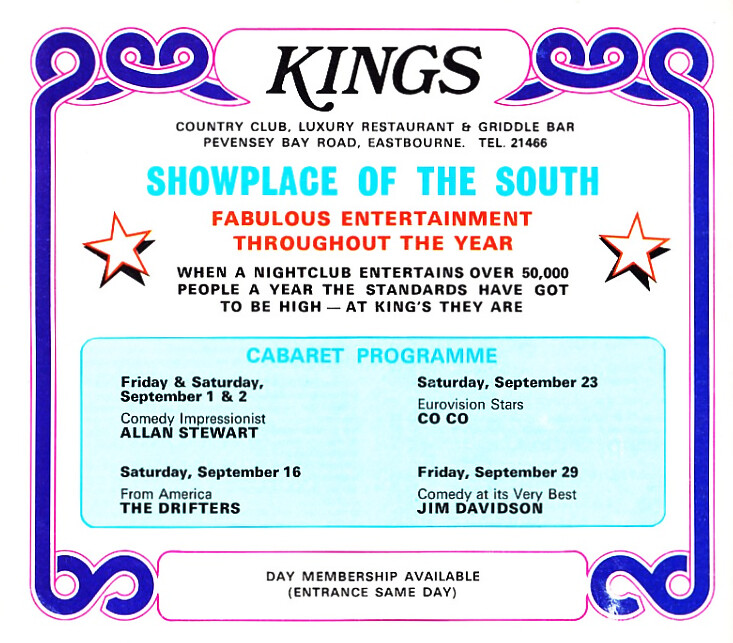The image is a vibrant and detailed advertisement for Kings, a luxury establishment located at Pavenzie Bay Road, Eastbourne. At the top, in large black letters, the name "Kings" is prominently displayed. Below this, smaller black text indicates it is a "Country Club, Luxury Restaurant, and Griddle Bar" with a telephone number 21466. The tagline "Showplace of the South" is written in blue text, followed by "Fabulous Entertainment Throughout the Year" in red. Centered beneath, in black letters, the statement reads, "When a nightclub entertains over 50,000 people a year, the standards have got to be high. At Kings, they are." Flanking this text are red and white stars, adding a flashy touch. The lower section features a blue-bordered area labeled "Cabaret Program," detailing upcoming events: Comedy impressionist Alan Stewart on September 1 and 2, The Drifters from America on September 16, Eurovision stars Coco on September 23, and comedian Jim Davidson on September 29. The very bottom of the image has a pink-outlined section that reads "Day Membership Available Entrance Same Day," emphasizing the accessibility and exclusive nature of the club. The overall design is colorful and eye-catching, lending a sense of luxury and excitement.